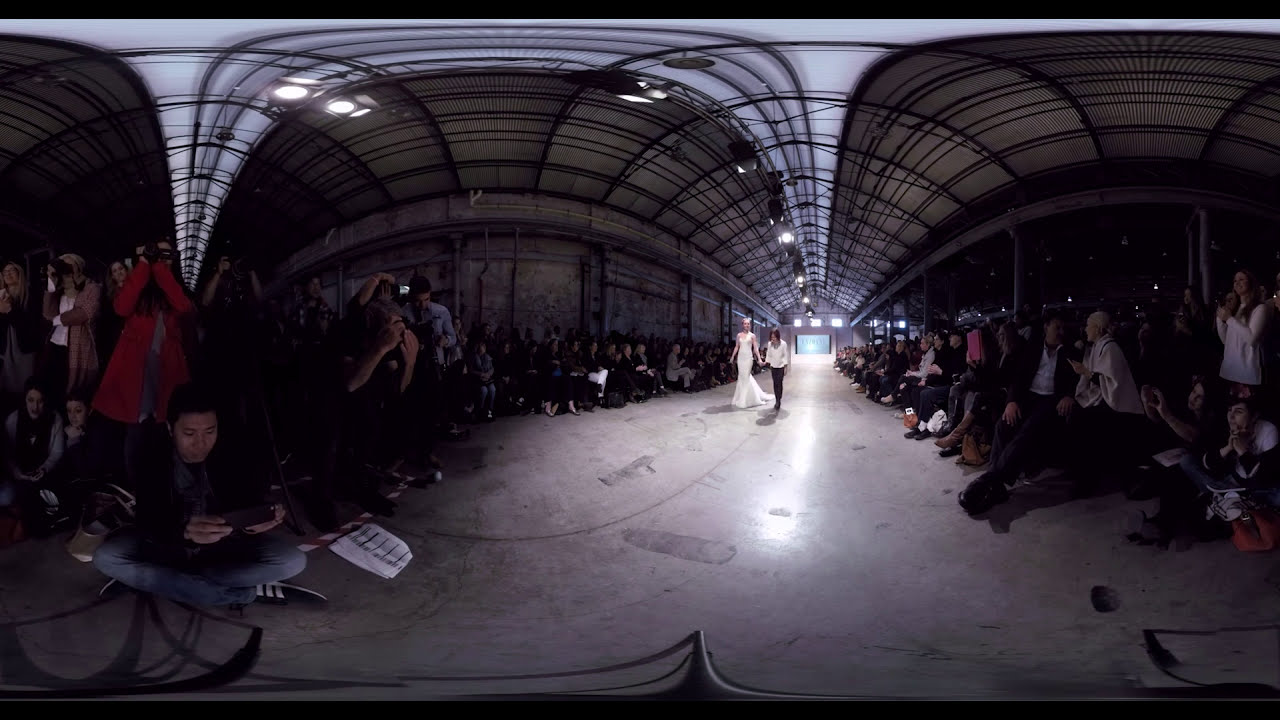The image depicts a somewhat distorted view, likely taken with a fisheye or 360-degree lens, of a large, open building complex resembling a long, warehouse-like hangar. The darkened scene is structured with a grid of scaffolding or girders supporting the roof, which is dotted with numerous spotlights. The walls are a dingy cream or brown color, and the floor appears to be cement. There are many people present, gathered on both the left and right sides of what looks like an aisle. It's possible that the event could be a wedding or a fashion show, supported by the presence of a woman in a long white gown walking down the central aisle. Accompanying her is a person wearing black pants and a white shirt. The audience, possibly numbering in the hundreds, is composed of individuals of varying ages, some seated against the walls and others standing while filming or taking photographs. Towards the front and in closer proximity, a man is seen sitting on the floor with his legs crossed, capturing the event on his phone. The entire scene is set against the backdrop of a dark, open night visible through large open doors at the far end of the room.